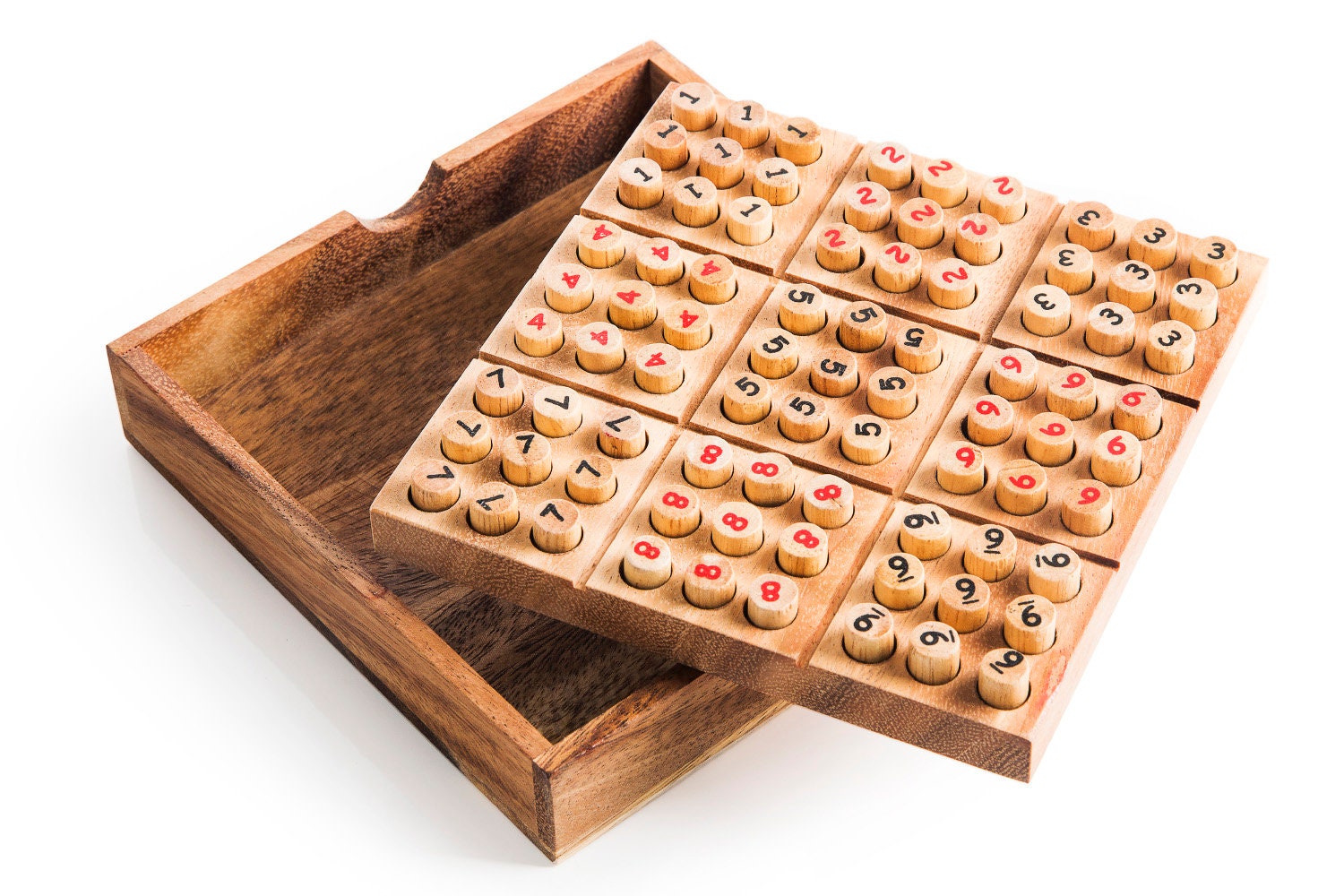The image depicts a detailed wooden tabletop game designed for a grid-based numerical challenge. This handcrafted game features a main square board that rests atop a hollow square wooden cabinet, emphasizing its dark and light brown tones. The game board is divided into nine smaller sections, each mirroring a tic-tac-toe layout with three rows and three columns. Each of these sections contains nine round pegs, organized in a grid format, and numbered from 1 to 9. The numbers are distinctly marked in black and red. The overall aesthetic, with its clean wooden construction and organized numerical arrangement, suggests a minimalist but engaging game, possibly presented as an advertisement highlighting its craftsmanship and strategic appeal.